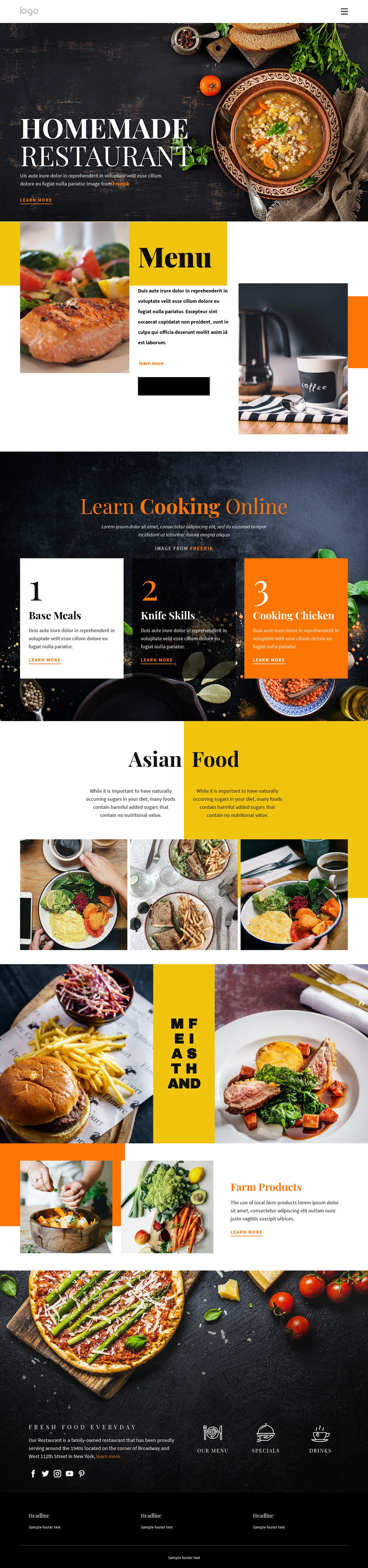The image features a prominently designed advertisement for a homemade restaurant with a black background. On the left side, the background is predominantly black, transitioning towards the right where a detailed plate of food is displayed, surrounded by various other food items and greenery. 

In the black area, there is white text that reads "Homemade Restaurant," with a lot of smaller text beneath it, mostly in white with some in orange, making it difficult to see clearly. To the right, there is a yellow rectangle labeled "Menu," adjacent to which is an image showcasing food along with a descriptive paragraph underneath in black, interspersed with yellow writing. 

Further to the right, there is an image of a coffee cup and a napkin with a small orange rectangle next to it. The entire background remains black with scattered food pieces, particularly visible towards the bottom. Text in white says "Learn Cooking Online" with more words underneath, mostly in white and some in orange.

A white rectangle marked "1" is visible, with mostly black writing underneath, transitioning to orange at the bottom. Nearby, a black rectangle labeled "2" in orange features white text beneath, ending in orange. Adjacent to this, an orange rectangle marked "3" in yellow has additional yellow writing underneath.

At the halfway point between left and right, a white rectangle labeled "Asian" is followed by more black writing. From this midpoint to the right, a yellow rectangle labeled "Food" features further text beneath it. Below this section are three images of food, followed by two more food pictures with a yellow rectangle in between containing indistinct writing.

Moving down, there is an orange rectangle with a food image partially overlaying it and another food picture beside it, featuring a mix of orange and black writing ending in orange. Towards the bottom left, a black rectangle showcases food items, likely a pizza on the left with tomatoes and jalapeno peppers. This is accompanied by mostly white text with a small portion in red, along with various small, indiscernible symbols in white.

This elaborate composition effectively highlights various food items and promotional text for the homemade restaurant, emphasizing their online cooking courses and diverse food offerings.